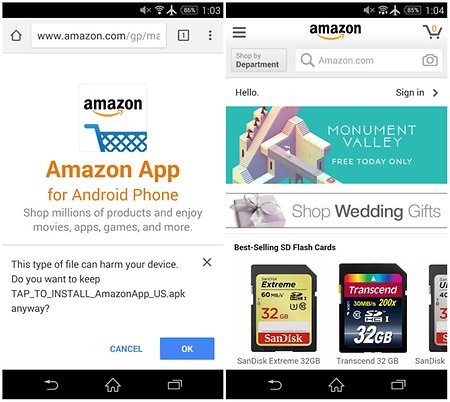**Caption:**

The image is a screenshot from the Amazon website, showcasing two adjacent sections. Both sections are set against a white backdrop with a thin black bar running horizontally across the top. 

In the top section of the primary image, the black bar contains several icons from left to right: a white sound icon with an 'X' indicating mute, a Wi-Fi signal strength icon, a blue airplane mode icon, a white box with the letters 'BEA' inside, and the current time displayed as '1:03'. The secondary image to the right mirrors the same setup but notes the time as '1:04'.

The upper left corner of the page features a home icon, followed by a URL in the search bar: "www.amazon.com/gp/ma...", which is truncated as it extends towards the right. To the right of the search bar are several icons: a white box with a black number one, a vertical ellipsis (three vertical dots), and a hamburger menu (three horizontal bars). Following a small gap, the recognizable Amazon logo in black with a yellow smile is displayed. At the far right is a black shopping cart icon with a yellow '0' inside it.

Beneath this, on the left side of the page, the Amazon logo is repeated in black with the yellow smile beneath it. A partial view of a blue shopping cart is visible in the center. Below this, yellow text reads "Amazon app," followed by "for Android phone" and "Shop millions of products and enjoy movies, apps, games, and more." Below this in black text is a warning message: "This type of file can harm your device." Subsequent lines read, "Do you want to keep," "tap_to_install_Amazon_app_US.APK," and then, "anyway?" with a question mark. Below this are two options: a blue "Cancel" button on the left and a blue "OK" box on the right.

At the top of the secondary image, "Shop by department" is written in black, above a search bar containing "Amazon.com" and a search icon on the left, with a camera icon on the right. Beneath this, on the left side, is a greeting, "Hello," and on the right, a sign-in prompt. Under this section, a green box shows "Monument Valley free today only" in white, accompanied by an image of MC Escher-like stairs in beige and purple hues. Below this is an image of a gray gift box with a ribbon, labeled "Shop wedding gifts." Lastly, three images of best-selling SD flashcards are displayed side by side, titled "best-selling SD flashcards."